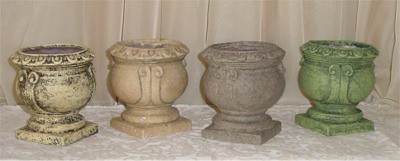This rectangular photograph, appearing as though it was taken with an older camera due to its slightly poor quality, captures a collection of four small, vintage-style ceramic planters arranged neatly on a white tabletop. The backdrop is a pleated brown curtain, giving a warm contrast to the white surface beneath. Each planter sits on a thin, square base leading up to a more ornate, filigree-patterned rim, suggesting an almost Roman design. The planters differ in color and slight markings, contributing to their antique aesthetic:

1. The leftmost planter is off-white with some black streaks, giving it a weathered look.
2. Next to it, a plain tan planter stands simply yet elegantly.
3. The third planter is a darker brown or taupe, contributing to the varied color scheme.
4. The fourth and final one is a vibrant jade green, adding a touch of brightness to the ensemble.

The planters' round bases and their narrowing then expanding shapes highlight their decorative intent, possibly intended for tabletop decoration or small plants. The photograph, small and narrow in dimension, emphasizes the rustic charm and antiquity of the planters, making them appear as though they could be perfect for an online listing or catalog.